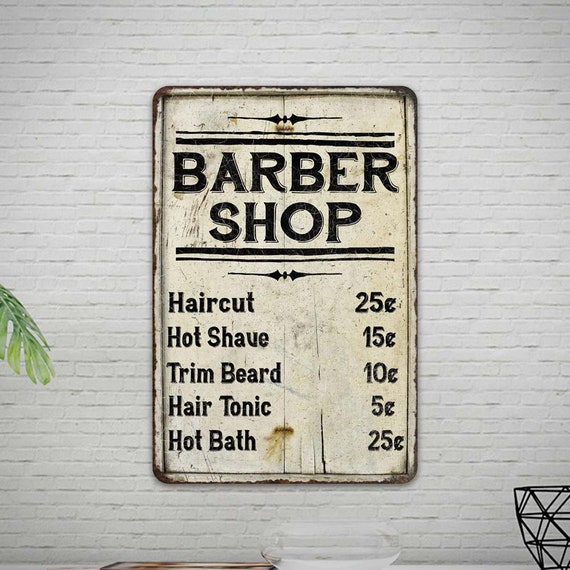This image features a mock-up promotional image of a vintage-style tin sign for a barbershop, designed to appear weathered and rusted around the edges with some rust stains and scratches in the center. The sign is mounted on a white brick wall. At the top of the sign, large black text reads "BARBER SHOP" in all capital letters, with "BARBER" positioned above "SHOP." The text is flanked by horizontal lines with small decorative triangles or border designs both above and below the inscription. Below this are listed various services and their prices in black lettering: Haircut for $0.25, Hot Shave for $0.15, Trim Beard for $0.10, Hair Tonic for $0.05, and Hot Bath for $0.25. The mock-up also includes a partial view of a table beneath the sign, on which sits a glass dish, along with a frond from a potted palm to the left, and a wire metal structure in the bottom right corner.